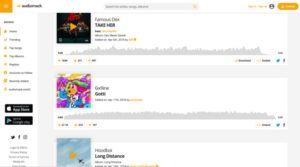The image depicts a pixelated screenshot of what appears to be a music website, likely resembling SoundCloud. In the upper left corner, there is an easily identifiable orange square next to some black text, which is unreadable due to the low resolution but presumably displays the website's name. The interface showcases three tracks. 

The first track appears to be titled "Time Her" and features a cover image with a black background and red text. Accompanying the track is a gray sound wave visualization line.

The second track's title begins with the letter "G" and features a vibrant cover image bursting with bright pink, blue, orange, and yellow colors. This track also includes a gray sound wave visualization line.

The third track seems to be titled "Long Distance" and has a cover image depicting the sky with an airplane in it. Like the others, it is accompanied by a gray sound wave visualization line.